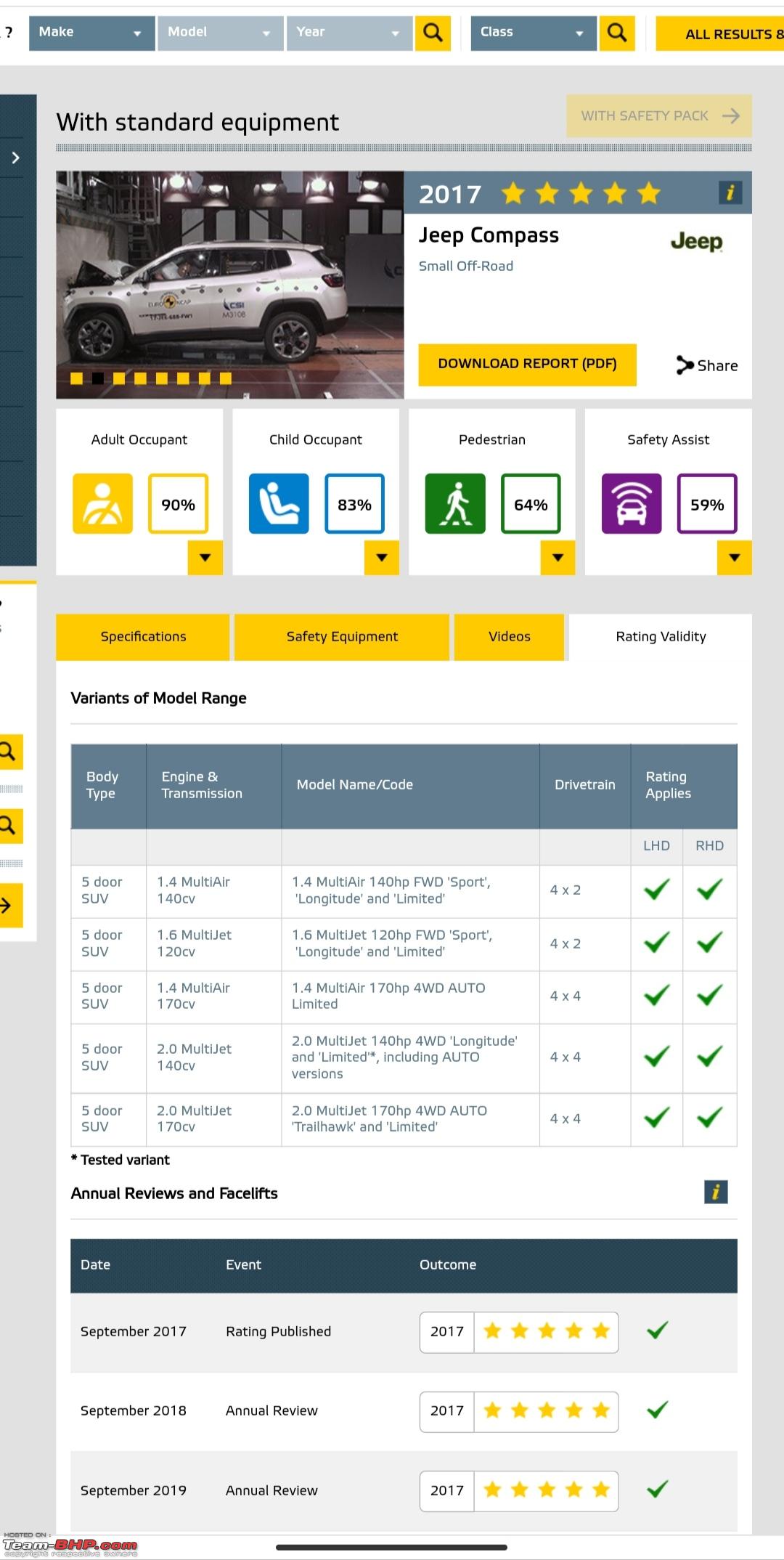The webpage prominently features an image of a white Jeep Compass near the top. The car is pictured facing the left side. Above the image are labeled blocks indicating "Make," "Model," "Year," "Class," and "All Results." The text "with standard equipment" appears, along with a header that reads "Jeep Compass" next to a button labeled "Download Report" in yellow.

Below the car image, there are percentage blocks with ratings: "Adult Occupant 90%," "Child Occupant 83%," "Pedestrian 64%," and "Safety Assist 59%." Following these, yellow blocks list categories such as "Specifications," "Safety Equipment," and "Videos," alongside a white box marked "Rating Validity."

Further down, the page provides information on "Variants of Model Range," highlighted by green headers for sections like "Body Type," "Engine and Transmission," "Model Name Code," "Drivetrain," and "Ratings." A column layout presents specific details under these headers. At the bottom, a green bar spans the width of the section, accompanied by dates and star ratings sorted by date.